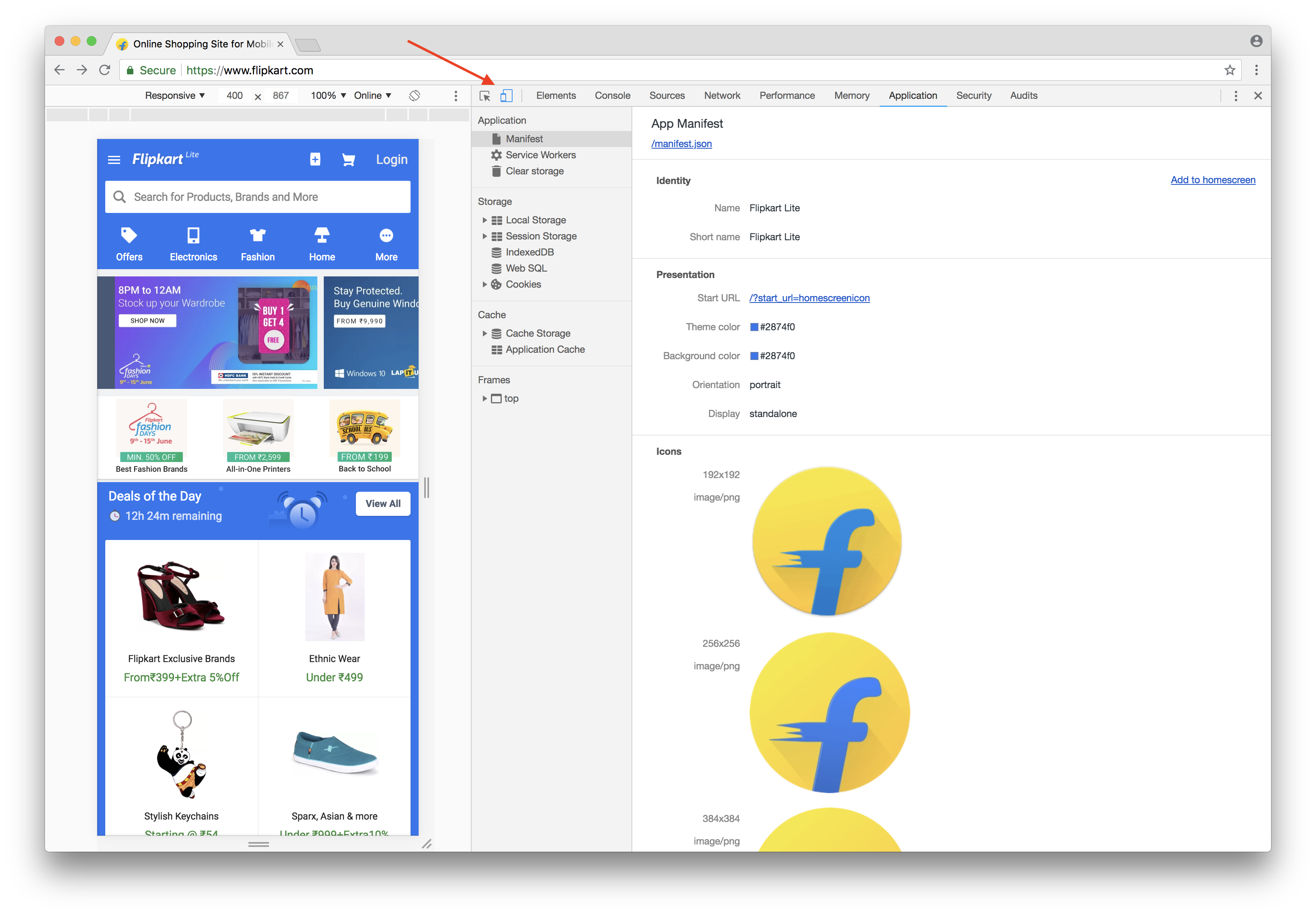This image is a screenshot of the online shopping site, www.flipkart.com. On the left-hand side, the Flipkart logo is prominently displayed in a blue box. Next to the logo, there are icons for a plus sign, a shopping cart, and a login option. A central white search box allows users to input queries. Below the search box, there is a navigation menu featuring categories such as Offers, Electronics, Fashion, Home, and More.

From 8 p.m. to 12 a.m., there is a special promotion encouraging customers to "stock up on your wardrobe" with a "Buy One, Get Four Free" deal. Additionally, there is a notice for a discount on genuine Windows software starting at 9,900 currency units (likely Indian Rupees).

Highlighted further are ongoing promotions like "Fashion Fairs" offering a minimum of 50% off on the best fashion brands from June 9th to June 15th. There are also deals on all-in-one printers starting from 2,599 currency units, and back-to-school supplies starting from 199 units. 

A 'Deals of the Day' section indicates that 12 hours and 24 minutes remain for these specials. Further promotions include Flipkart exclusive brands starting from 399 units plus an extra 5% off, ethnic wear under 499 units, and stylish keychains. Shoes from brands like Sparks and Asian are offered under 999 units with an additional 10% off. 

On the right side of the screen, there’s an app manifest for the Flipkart mobile app, detailing information about the app's identity, short name ("Flipkart"), and presentation details like the start URL, home screen icon, theme color, background color, orientation, and display format. The manifest also includes three different-sized icons featuring a circular design with a yellow background and an 'F' symbol adorned with flares emanating from the crossbar of the 'F'.